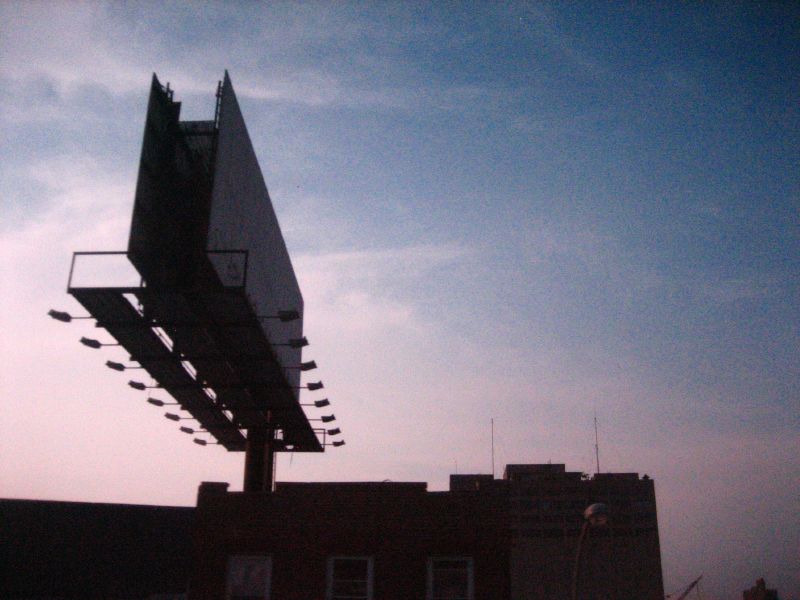This outdoor photograph, taken at an upward angle, captures a billboard set against a serene bluish-pink twilight sky. Positioned towards the left side of the frame, the billboard consists of two rectangular panels separated by a dark central object. The base of the billboard features several small lights mounted on thin stems, adding a distinctive detail to the structure. Below, the roofline of a building extends across the bottom of the image, occupying about four-fifths of the frame and anchoring the scene in an urban environment.